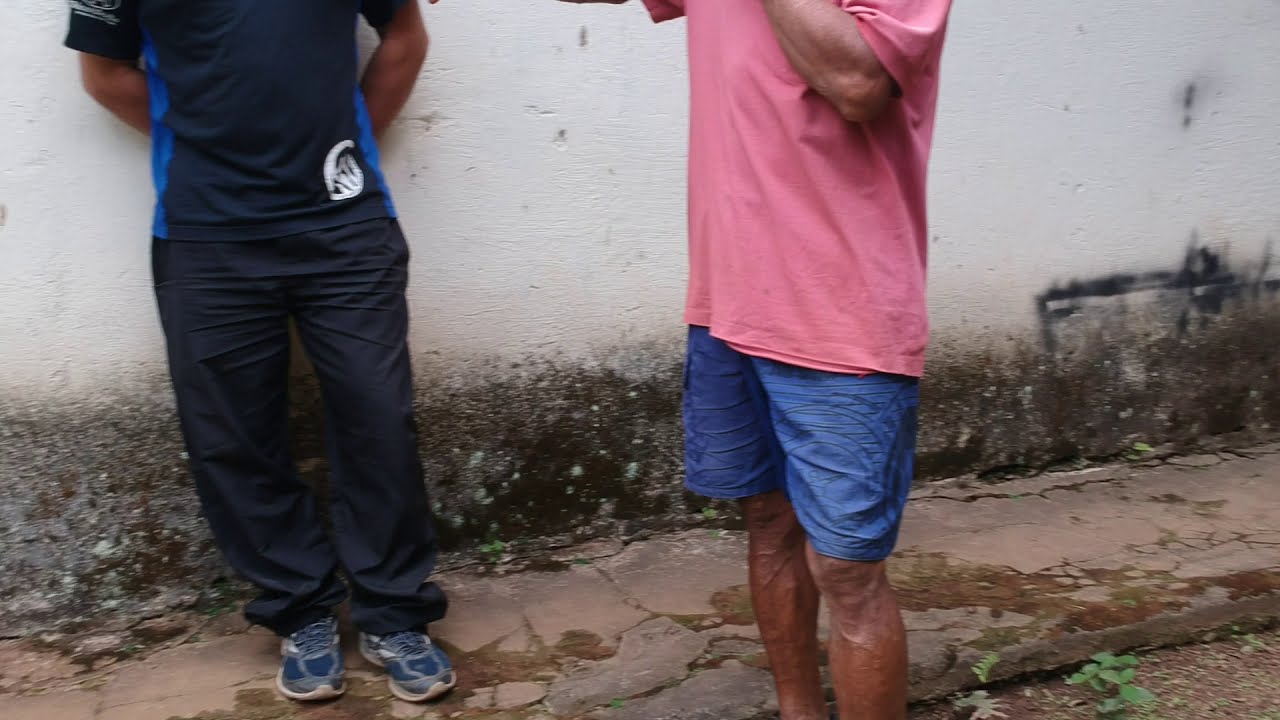The image features two men standing outside against a white wall that appears weathered and stained with patches of dirt and grime towards the bottom. The ground beneath them is a cracked, worn-out sidewalk interspersed with orange tiles, some dirt, and sprouting weeds, suggesting it might have recently rained. The man on the left, leaning against the wall with his hands behind his back, is dressed in a dark blue shirt with light blue streaks along the sides, dark blue pants, and blue sneakers. His visible arms extend from the elbows down before they go behind his back. The man to his right is wearing a pink t-shirt and blue shorts, with his tanned legs visible. Though his feet aren't shown, one of his elbows is raised as if his hands are reaching towards his face. The scene depicts a rough, somewhat run-down environment.